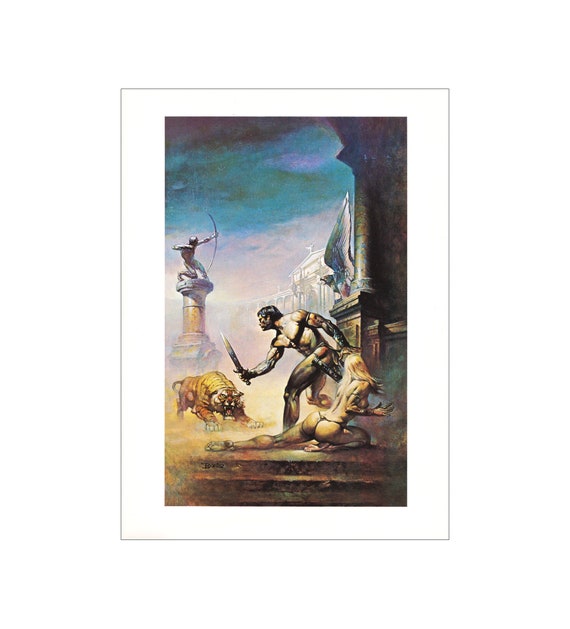The painting depicts a dramatic ancient battle scene, likely inspired by Roman times. Centered in the foreground, a topless man clad in white brandishes a short sword, facing off against a menacing tiger poised to pounce. Near him, a frightened woman kneels on the ground, looking away from the impending danger. The background showcases a classic ancient building facade, accompanied by a column crowned with a statue of an archer aiming towards the heavens. Another column, partially visible on the right side of the image, appears to support a sculpture that seems to resemble a griffin. The sky above is filled with dark, foreboding clouds, enhancing the tense atmosphere of the scene. The color gradient of the sky shifts from a light peach to deep blue-green hues. This intense and evocative composition suggests a gladiatorial scene or an ancient battle, capturing the viewer's imagination and placing them right in the midst of the action.